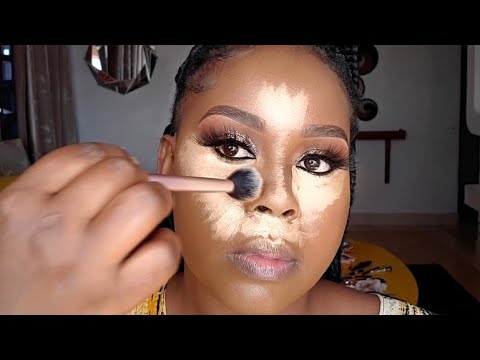The image depicts a younger Black woman with tightly curled black hair on one side, facing the camera as she applies makeup. She uses a brush with a wooden handle and black bristles to dab silvery-white makeup around her nose, upper cheeks, and beneath her nostrils. Her eye makeup is already elaborate, featuring glittery, smoky taupe eyeshadow and large false lashes that complement her cut eyebrows. Notably, there's a splotch of makeup above her painted eyebrows and on her nose. She appears to be filming a makeup tutorial, likely for YouTube, as she expertly demonstrates the highlighter application technique. Her skin, flawless aside from the unblended makeup, basks in a gentle light. The background showcases a white wall adorned with an octagonal silvery mirror. Her hand is slightly out of focus in the foreground, emphasizing the intricate process of her beauty regimen.